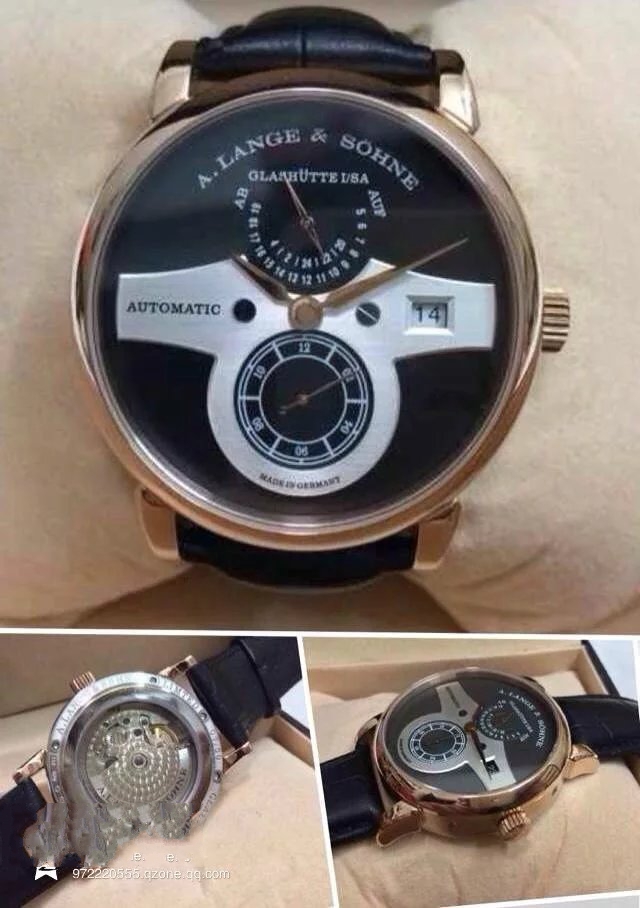This image collage features a luxurious wristwatch, presented in three distinct views. The top image showcases the watch elegantly draped over a white pillow, highlighting its sophisticated design. The timepiece boasts a genuine leather strap and a striking rose gold exterior. Its black face is beautifully contrasted by white accents and lettering, prominently displaying the brand name "A. Lange & Söhne." The watch face is adorned with delicate rose gold hands and includes a couple of intricate sub-dials, though the absence of numerals makes the time slightly challenging to decipher. Notably, the watch is crafted in Germany, a detail proudly inscribed on the dial.

The bottom half of the collage is split into two images, offering alternate perspectives. On one side, the intricate mechanics of the watch’s backside are visible, revealing the precision engineering within. The other side provides a side view, accentuating the watch’s sleek profile and craftsmanship. This trio of images collectively underscores the timepiece’s elegance and engineering excellence.